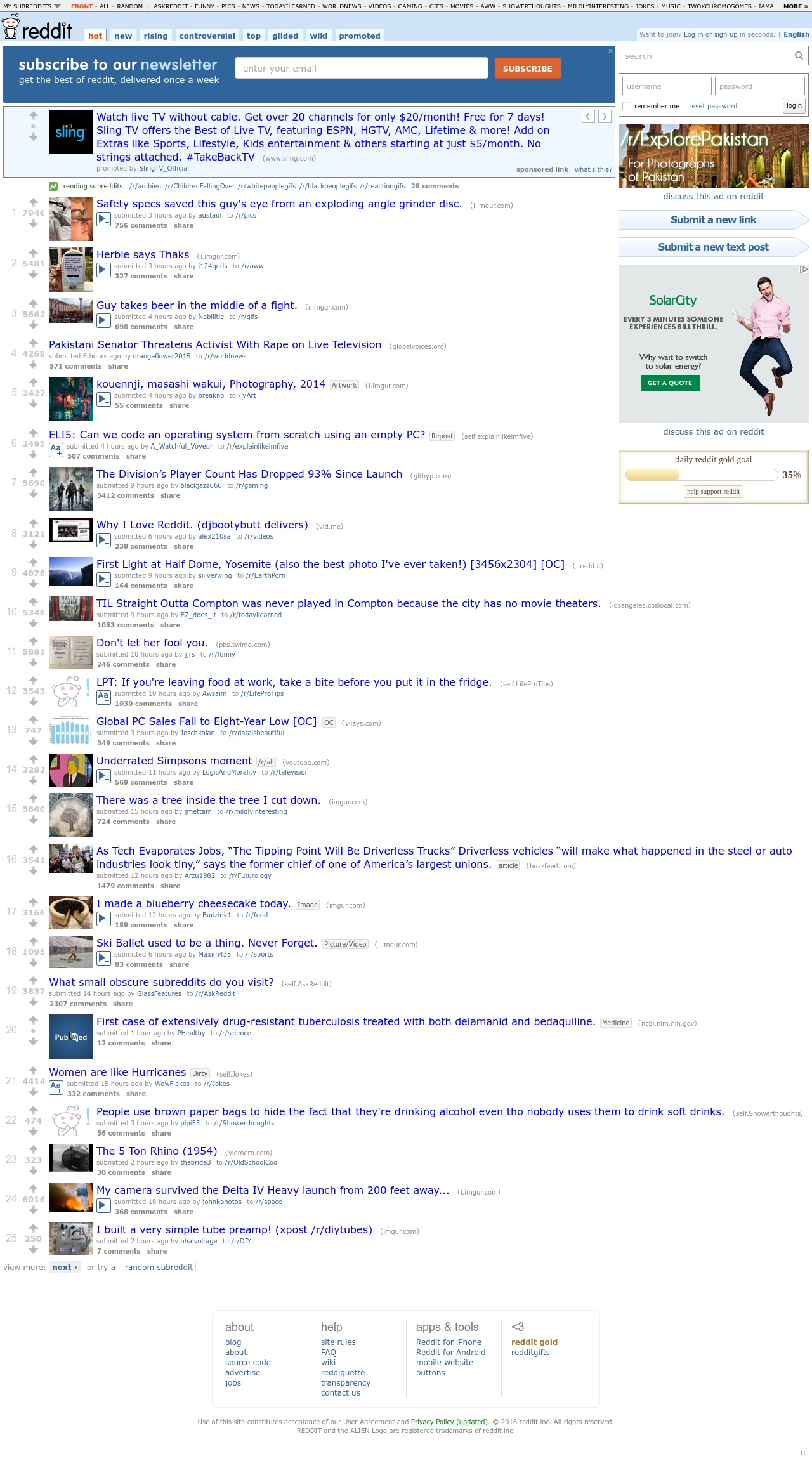This screenshot, originating from Reddit's early 2010s interface, showcases the platform's older design, likely from around 2009 to 2010. The image quality is low and the details are tiny, making text nearly unreadable. In the top left corner, we can observe the classic Reddit logo, characterized by lowercase black letters and the vintage white Reddit avatar without a red circle background. The header sports a light sky blue backdrop, beneath which lies a medium blue rectangle inscribed in white text that reads, "subscribe to our newsletter." Adjacent to this is a large white field intended for email addresses and a small, square, orange submission button to its right. The left section of the page displays a list of stories and headlines, though the text and accompanying images are too small to discern. On the right side, there's an advertisement against a gray background, featuring a man in a white T-shirt and black skinny jeans, appearing to leap mid-air.